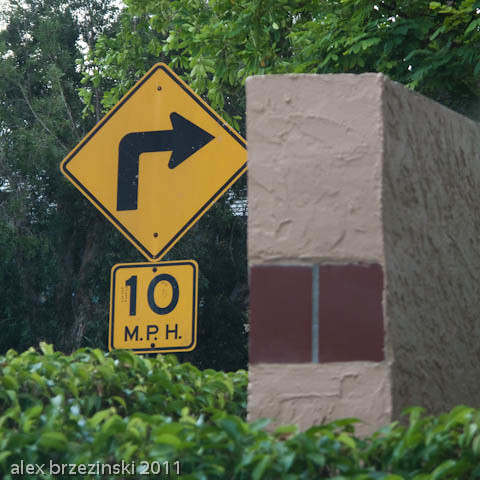This color photograph captures a detailed scene featuring a vertical, textured concrete structure with two small, vertical red rectangles and a bluish line in between them on its front. To the left of this structure stands a prominent diamond-shaped, yellow street sign with a black arrow pointing upwards and then to the right. Beneath the sign, a square yellow and black box displays "10 MPH" in bold black letters. The background is rich with greenery, including numerous trees and various plants and bushes surrounding the structure, providing a lush, natural setting. The wall, primarily grey concrete, has some sections described as light brown or beige stucco and features a reddish area near the bottom. In the bottom left corner, discreet text reads "at Alex Brzezinski, 2011." There are no people, animals, or motorized vehicles in this serene outdoor scene.